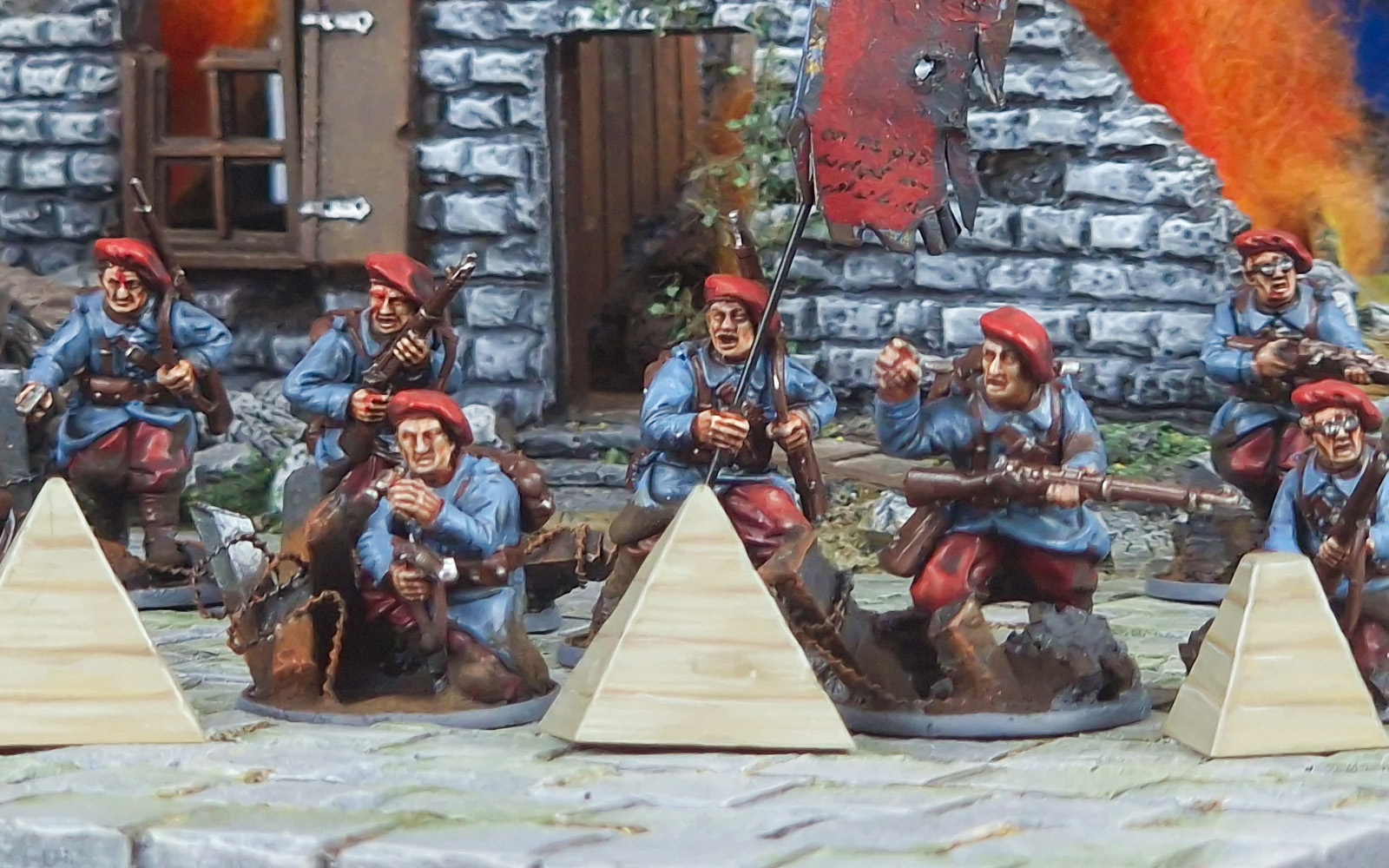This is a highly detailed, close-up photograph of a diorama featuring metal miniature figures that represent southern European military men from the early 20th century. There are seven to nine figures, each dressed in a distinctive uniform consisting of red berets, blue jackets, red pants, and boots. These soldiers, who appear to be either Italian or Greek, are armed with brown wooden single-shot rifles and are depicted in various action poses, as if engaged in battle. The scene is set on brick cobblestones, in front of a partially damaged stone house with a wooden door. Flames suggest the aftermath of a recent explosion, adding to the realism of the scene. Small pyramidal defensive structures are positioned in front of the soldiers. The background includes a torn red flag with unreadable text, contributing to the wartime ambiance. Despite some figures having duplicate faces, the overall depiction is lifelike and dramatic, capturing a moment of intense conflict.